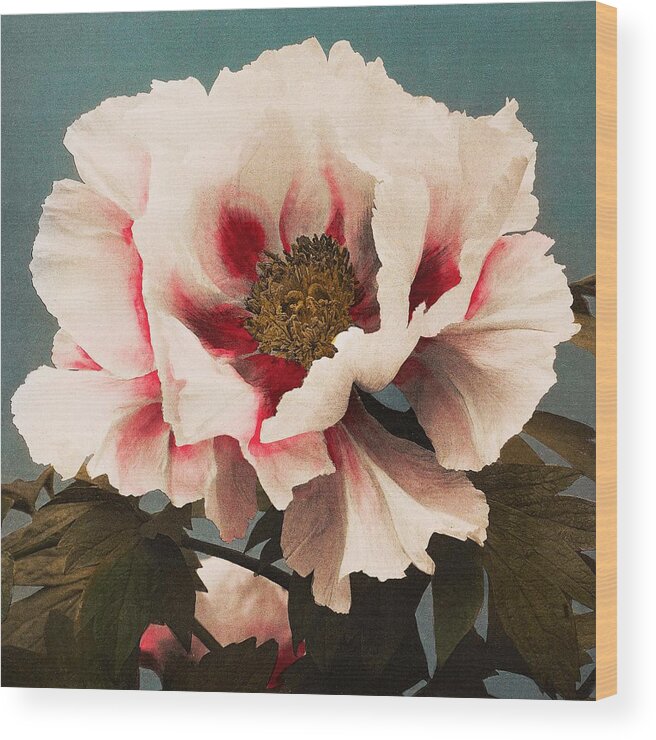This image shows a highly detailed painting on what appears to be a wooden canvas, capturing a large, striking flower as the focal point. The flower's petals are predominantly white, with the color transitioning into shades of bright pink and deep red as they approach the center. These large, flowy petals frame the intricate middle section, which features a blend of yellowish-green and brownish tones, possibly representing the stamen or seeds. Surrounding the flower's base are dark green leaves, with their rich, olive hues contrasting against the flat teal background. The wooden canvas, slightly tilted to reveal unpainted wood grain on the right side, adds a unique texture and depth to the artwork. The combination of these elements creates a visually compelling and vibrant composition.